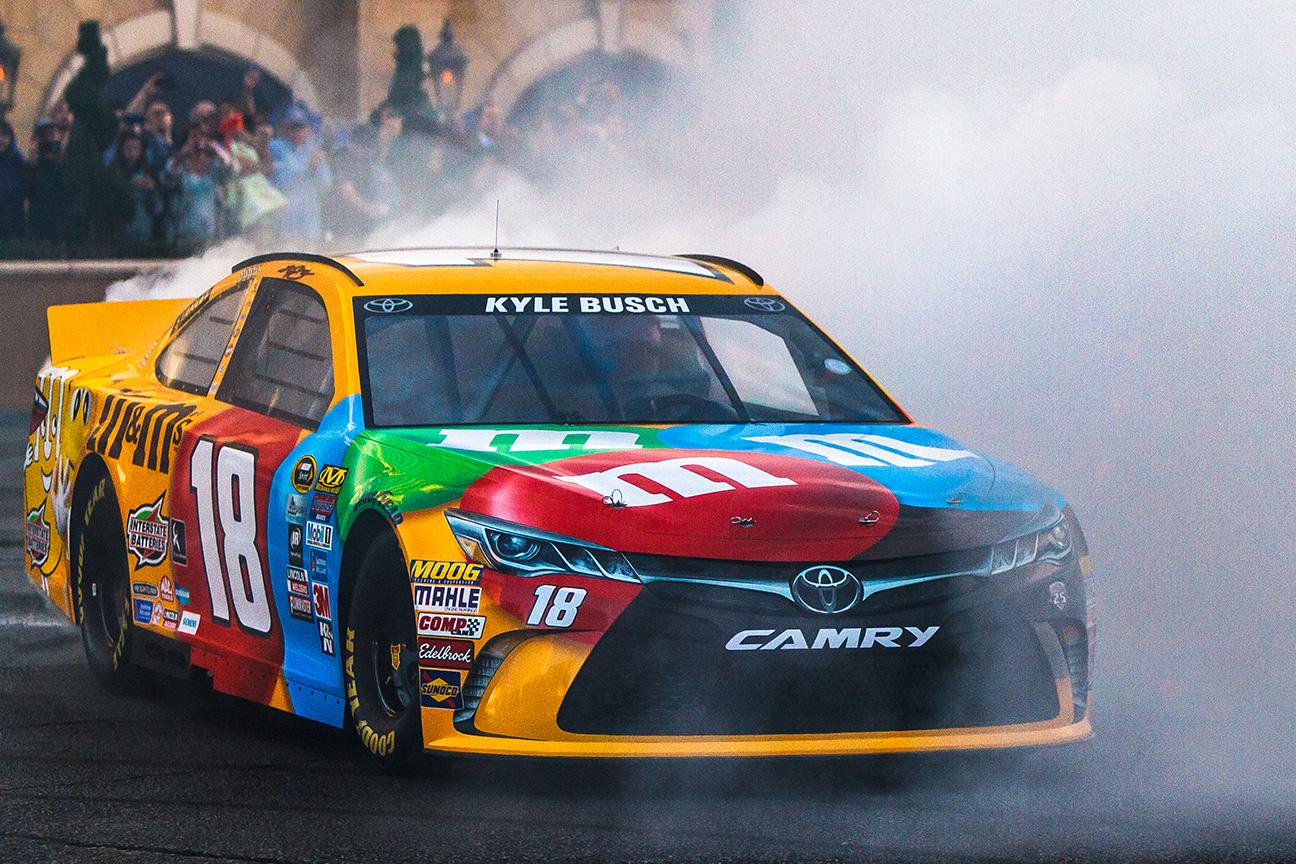The image captures an exhilarating moment of a NASCAR race car performing a burnout, leaving a trail of thick smoke behind and to the right as it skids against the black asphalt. The race car, primarily yellow, is adorned with colorful, enlarged M&M candies prominently featuring green, red, and blue ones on the hood, each marked with the distinctive white lowercase "M." The front of the car showcases a stylized bull's head logo encircled, along with "Camry" inscribed on the grille. The car's left side boldly displays the number 18 in gigantic white characters. The background reveals a crowd of cheering spectators in front of a tan stone building with symmetrical white stone arches. The car is covered with various brand stickers and advertisements, with "Kyle Busch" visibly written atop the windshield. The car’s black Goodyear tires, including yellow writing, add to the detailed depiction of this triumphant scene.